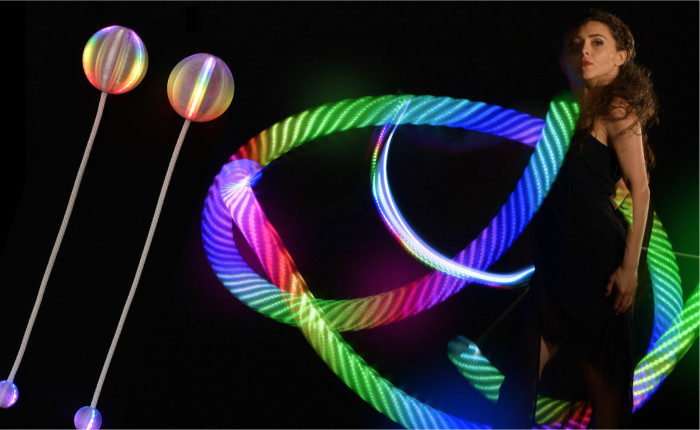The image captures a woman in a black strapless dress with brunette hair styled in a curly ponytail cascading over her shoulder. Her skin appears Caucasian, and she has striking red lips, adding to her serious expression as she looks directly at the camera. Positioned on the right side of the frame, she stands against a pitch-black background, giving the impression that she has been photoshopped into the scene. Surrounding her are vibrant, neon-like lights that create a surreal and enchanting atmosphere.

In the center of the image, a large, swirling object resembling a twisted rope is illuminated in a spectrum of rainbow colors—red, orange, yellow, green, blue, purple, and indigo. Further enhancing the fantastical setting, the left side of the image features two rod-shaped structures, each ending in spherical lights that echo the rainbow hues found in the central swirl. These spheres, reminiscent of lollipops, have translucent qualities with intricate patterns of greens, yellows, and purples, adding depth and color to the overall composition. The blending of the woman's poised stance and the vivid, almost otherworldly lighting elements creates a captivating and vivid scene.